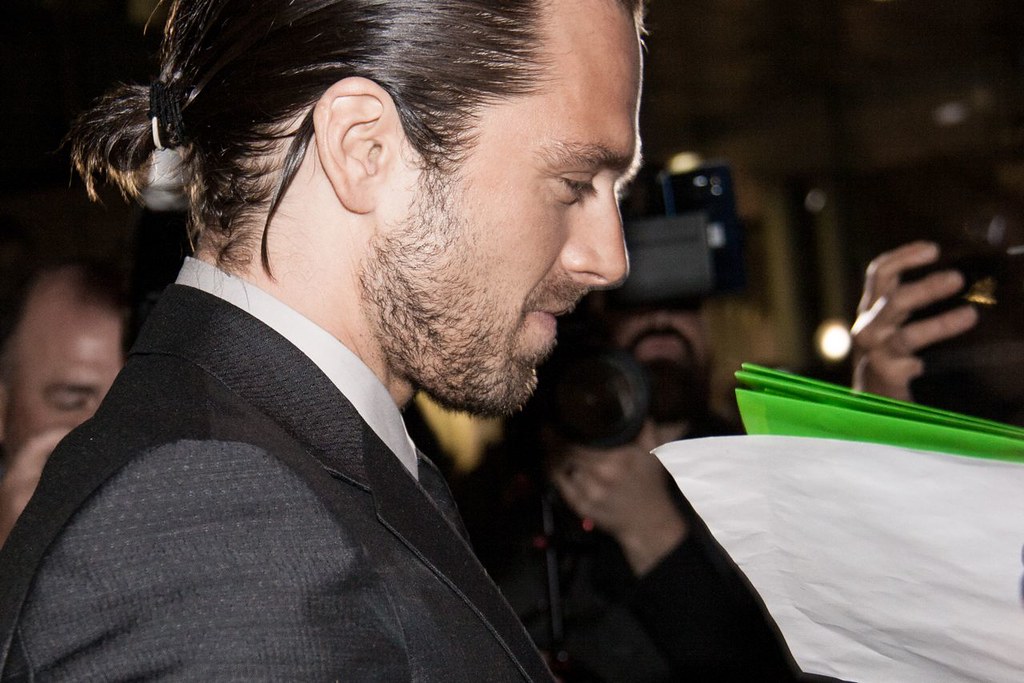This color photograph features a man with slick, shiny dark hair pulled back into a small ponytail, positioned on the left side of the frame. He is dressed in a gray dress jacket with a white shirt and a dark tie. The man, gazing slightly downward to the right, sports a closely shaved beard that appears like a growing shadow, indicating it is either trimmed that way or simply not freshly shaved.

Behind him, several photographers are visible, aiming their cameras toward him and to the right. The background is predominantly dark, creating an ambiguous setting that could be the interior or exterior of a building, though illuminated lights are subtly visible in the distance.

The bottom right corner of the image is occupied by a person holding what appears to be a green folder containing white papers. This element adds a hint of context but remains secondary to the central focus of the man being photographed.